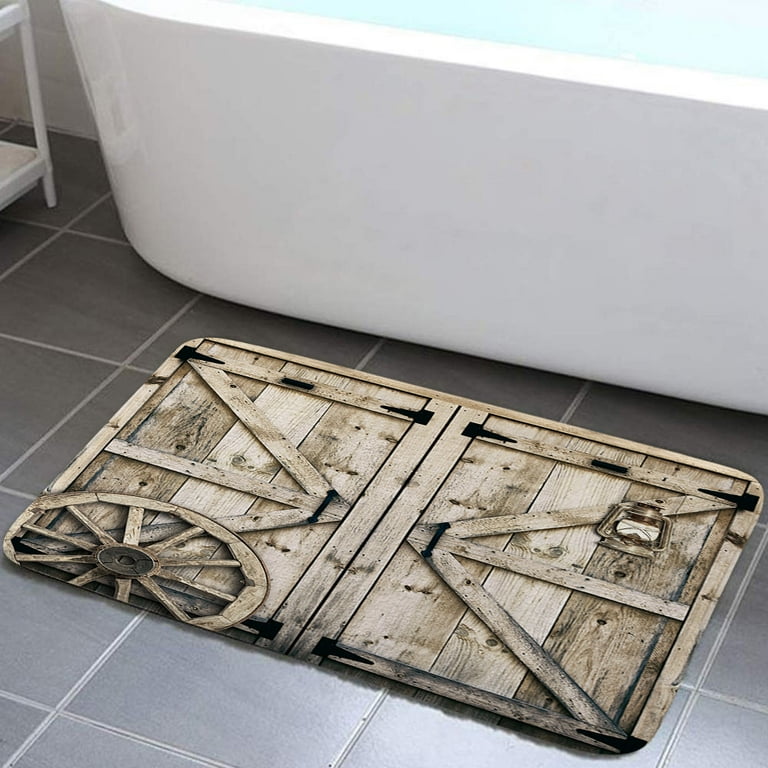The image depicts a detailed and intriguing bathroom scene. The floor of the bathroom features simple, gray tiles leading up to a white bathtub located at the upper right-hand side of the frame. The bathtub appears to be filled with water that gives off a teal blue hue, possibly due to the lighting, and there's a partially visible white shelf unit to the left.

The focal point of the image is a unique bath mat designed to resemble a pair of rustic wooden barn doors. The bath mat is composed of natural weathered-looking wood in tan and brown shades, and each half of the mat displays traditional barn door cross marks. The two segments of the mat also feature black hardware elements, such as hinges. Three wooden rods protrude from the center of each side, adding to the authentic barn door appearance.

Additionally, there are two distinctive props enhancing the barn door illusion: the left segment of the mat is adorned with a large, old-fashioned wagon wheel made of wood, and the right segment is accessorized with an antique-looking gas lantern hanging from it. These elements combined create a visually striking and imaginative interpretation of a bathroom setting.